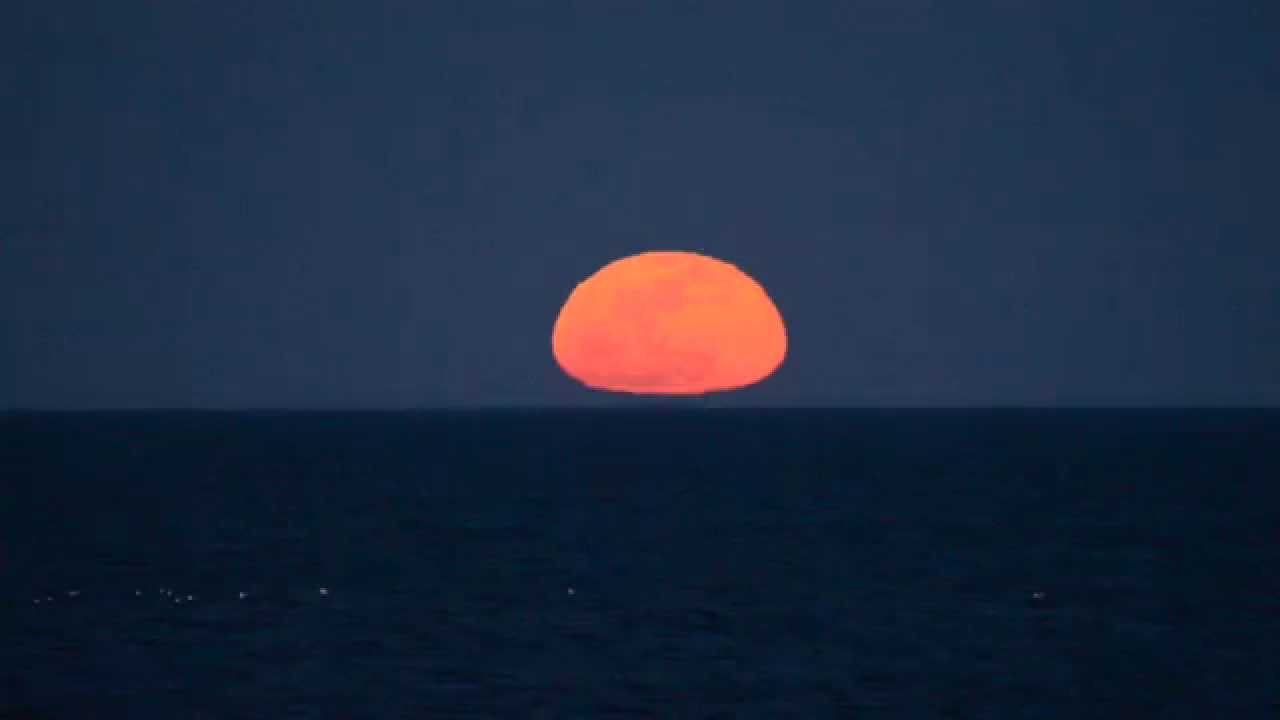This color photograph, captured in landscape orientation, vividly depicts a sunset over the ocean. The lower half of the image is dominated by very dark, almost black water, with faint ripples tinged with a slight white froth, set against a dark navy blue backdrop. The upper half transitions into a medium-tone dark blue sky, nearly merging with the dark waters below. Central to the composition is the sun, appearing as a bright orange orb, its shape somewhat elliptical with a flattened bottom, reminiscent of a sunny side up egg. The sun hovers just above the horizon, illuminating the sky as it reaches the final moments before sinking completely out of sight. The overall scene evokes a realistic and serene portrayal of a coastal sunset, with an emphasis on the contrasting colors and the tranquil yet imminent close of the day.